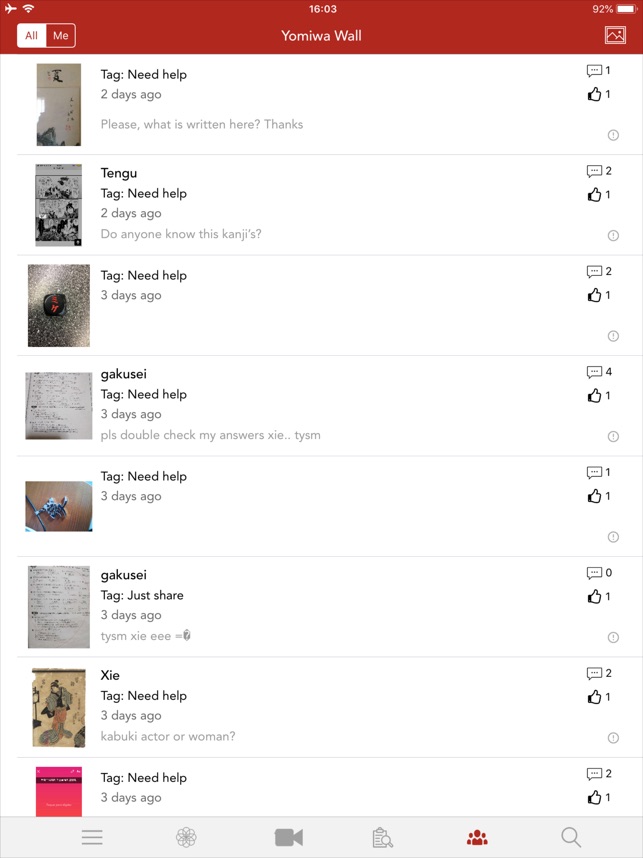This image is a screenshot of a website displayed on a tablet, as indicated by its larger size compared to a phone. At the top of the screen, the device is in airplane mode, connected to Wi-Fi, and the time is 16:03 (4:03 PM). The header of the webpage reads "Yomiwa Wall," and the battery is at 92%. There is also a picture emoji alongside labels "All" and "Me," with the "All" section currently displayed.

The content consists of eight different posts. Each post features a photograph and various user interactions:

1. **Post 1**:
   - Photo included.
   - Tag: "Need help".
   - Posted two days ago.
   - Text: "Please. What is written here? Thanks."
   - 1 thumbs up and 1 comment.

2. **Post 2**:
   - Photo included.
   - Tag: "Need help".
   - Posted two days ago.
   - Text: "Do anyone know this kanjis?"
   - 1 thumbs up and 2 comments.

3. **Post 3**:
   - Photo included.
   - Tag: "Need help".
   - Posted three days ago.
   - 1 thumbs up and 2 comments.

4. **Post 4**:
   - Tag: "Need help".
   - Posted three days ago.
   - Text: "Please double check my answers. X-I-E. Thank you so much."
   - 1 thumbs up and 4 comments.

The bottom of the screen features four additional lines, which are not fully visible in the provided description.